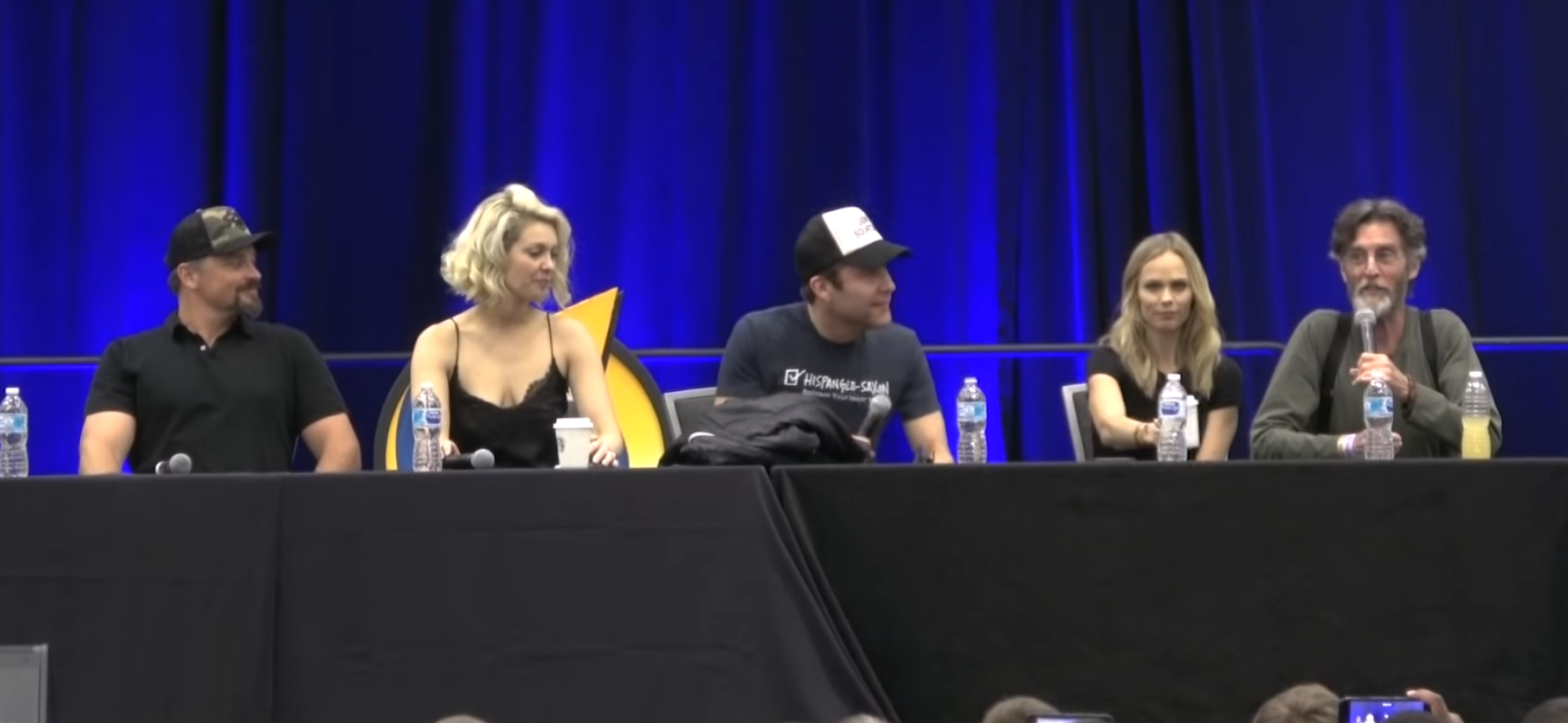In the image, five individuals—three men and two women, all of whom are white—are seated at a large conference table draped with a black cover, situated on a stage. They appear to be participating in a panel discussion, likely at a convention. The backdrop features bright blue curtains, enhancing the professional setting. Each panelist has a water bottle and a microphone in front of them. The men include two who are wearing hats and beards, and one older man without a hat, sporting long grey hair. As they engage with their audience, most of whom are out of frame except for a few visible in the front, the panelists are all facing forward, with some glancing to their left, presumably listening to the older man on the far right, who holds a microphone and seems to be speaking. The outfits of the panel members are predominantly black, white, or dark gray, maintaining a cohesive and formal appearance.